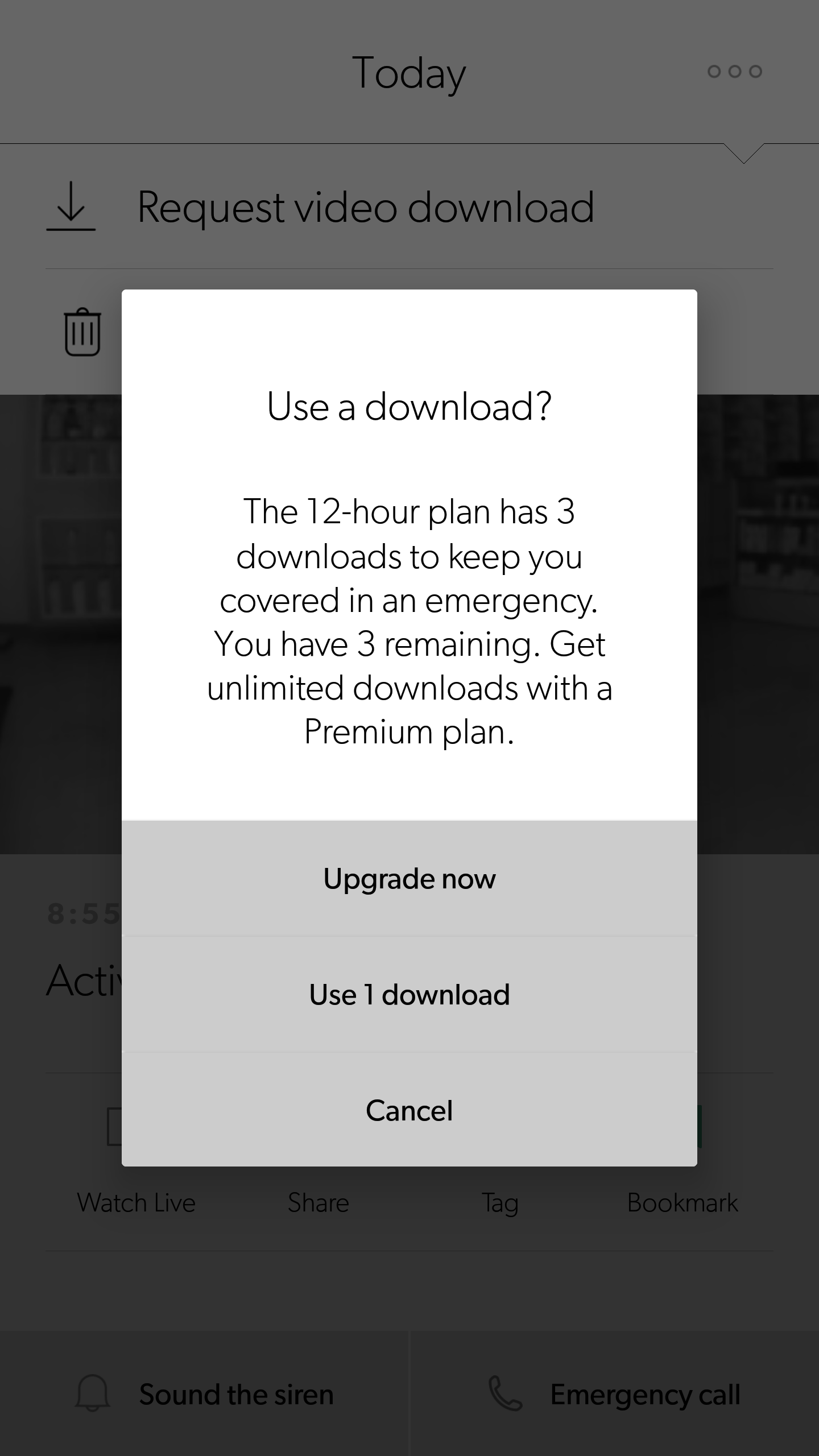This image is a screenshot of a download page featuring a prominent pop-up notification in the center. The pop-up's design is split, with a white top half and a gray bottom half. At the top of the pop-up, bold text states, "Use a download." This is followed by an explanation of a "12-hour plan" that offers three downloads for emergency use, with a note that "You have three remaining." A prompt below this offers to "Get unlimited downloads with the premium plan."

Under the text, three gray buttons are stacked vertically, labeled "Upgrade Now," "Use One Download," and "Cancel."

In the background, towards the top of the page, there is a section labeled "Today" situated beneath three vertical white dots located in the upper-right corner. Below this, text reads "Request video download," accompanied by a download icon featuring a down arrow to its left. Further down, an item labeled "L1" has a trash can icon adjacent to it.

The entire layout emphasizes the call to action for either utilizing the available downloads or upgrading to a premium plan for unlimited access.